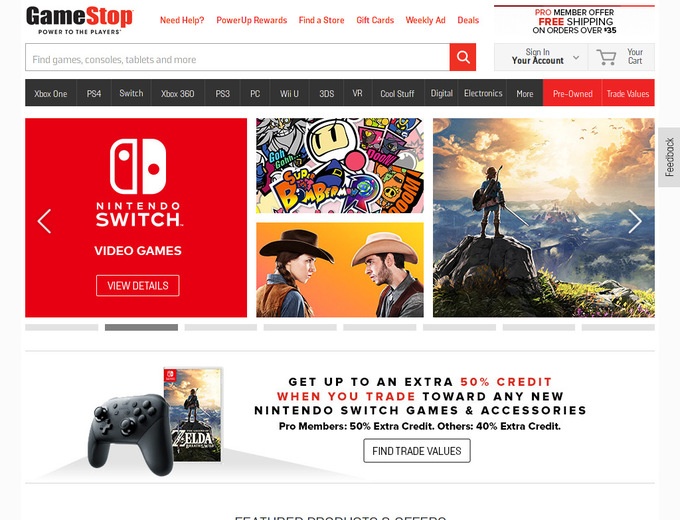In this vibrant screenshot of a GameStop store, a lively scene unfolds featuring various gaming elements. At the center, players are engrossed in a multiplayer game on a Nintendo Switch, surrounded by shelves filled with a wide assortment of video games. Prominently displayed are multiple Redbox machines, brimming with rental options. To the right, an amusing image captures a little cowgirl and cowboy facing each other against a whimsical background. Above them, an anime poster adds an artistic flair, while to the left, a man peers over into the crowded area.

Exciting promotional offers are highlighted throughout the store. Customers can receive up to 50% extra credit for trading in new Nintendo Switch games and accessories, and 40% extra credit for other trade values. At the top of the scene, a bar labeled "Need Help?" provides guidance and features icons for PS4, Switch, Xbox 360, PS3, and Wii U systems. The store is buzzing with an enthusiastic atmosphere, promising great deals and a wide range of gaming products.